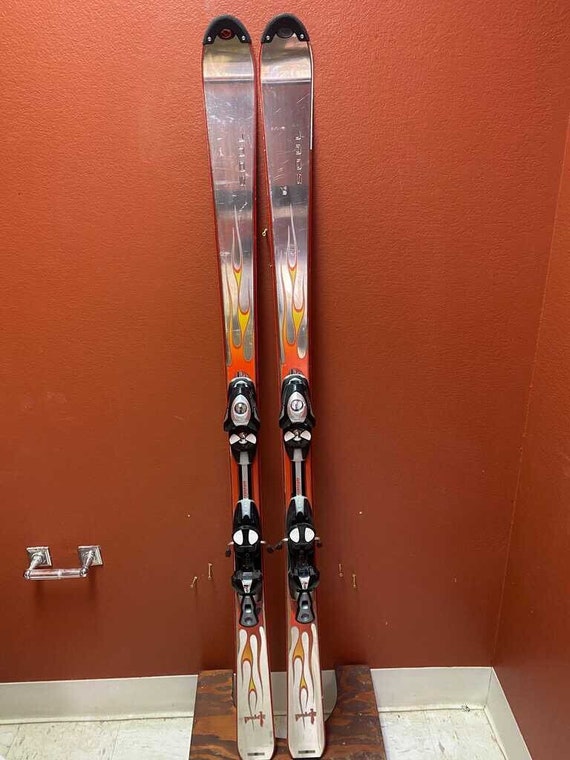This image depicts a pair of skis propped against a red-painted wall, in what appears to be a bathroom. The skis, measuring approximately four and a half to five feet in height, feature a polished metal body with striking red, orange, and yellow flame designs. The top of the skis showcases a carved brand name, which is not legible, and the tips are reinforced with black plastic plating. The skis are positioned on a small wooden structure or stool. To the left, a silver metal toilet paper holder is mounted on the wall, though it lacks a roll of paper. The bathroom floor is white tile with a slightly dirty appearance, and white cove base trim lines the base of the walls. This eclectic scene suggests the skis might be drying in this unusual storage location.